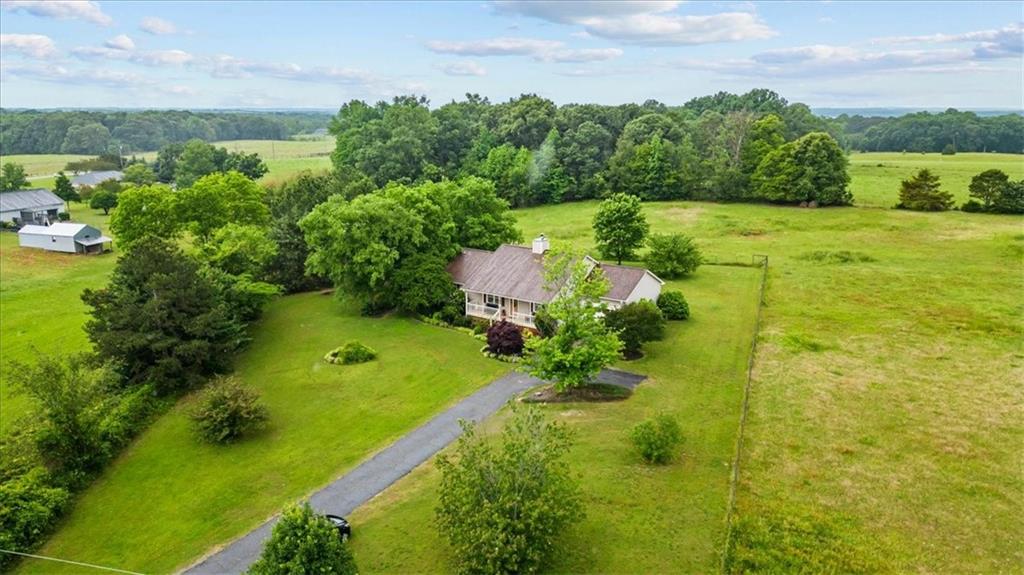This image captures a picturesque rural scene from a high vantage point, possibly from a helicopter. At the center is a charming white house, most likely a single-story, nestled within a vast, vividly green field. The foreground features a long driveway leading up to the house, bordered by freshly cut grass. Surrounding the house are numerous deeply green trees, extending into the distance where the horizon is lined with more trees as far as the eye can see. To the left of the house, there are a couple of additional structures, perhaps sheds, a mobile home, or a barn with a tin roof. The blue sky above is dotted with sizable white clouds, enhancing the serene atmosphere. A few telephone lines are subtly visible, outlining the expanse of the property. Overall, the dominant green of the grass and trees commands immediate attention, while the scattered buildings and sky create a tranquil, idyllic countryside setting.